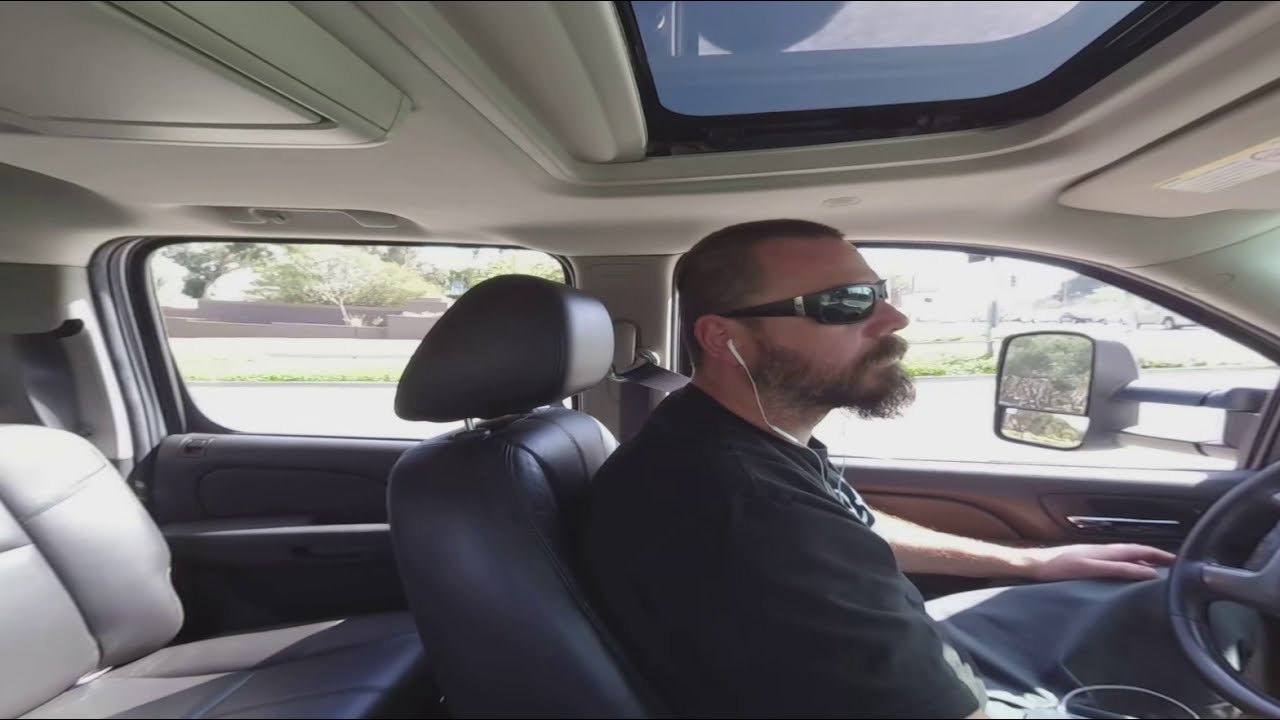A middle-aged Caucasian man, likely in his 40s or 50s, is sitting in the driver's seat of a spacious car, possibly an SUV. The vehicle's light beige interior features modified leather seats, a dual moon and sunroof with the front portion retracted to reveal the glass, and rolled-down windows on the driver’s side. Wearing black sunglasses and white wired earbuds, the man sports a scraggly, unkempt beard and mustache, along with short buzzed black hair. He is dressed casually in a black t-shirt and jeans. With his left arm resting over his knee and both hands away from the steering wheel, it implies the car is stationary. The background reveals a suburban street lined with trees and bushes. The lighting casts shadows across the driver's seat, adding to the man’s stressed or possibly angry demeanor.